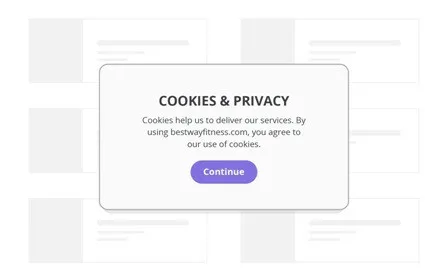Screenshot from Bestway Fitness Website Featuring a Cookie Consent Pop-up Window

In this screenshot from the Bestway Fitness website, the focal point is a pop-up window titled "Cookies and Privacy." The window, distinguished by its light gray border and rounded corners, contains a detailed message. The description within the window reads: "Cookies help us to deliver our services. By using bestwayfitness.com, you agree to our use of cookies." Below this informative text, there is a prominent "Continue" button in a striking purple color, also featuring rounded corners to complement the window’s design.

In the background, partially obscured by the pop-up, is a grid layout that appears to be part of the main website interface. This grid consists of alternating gray and white rectangles, acting as placeholders for content, with some rectangles containing small horizontal lines suggesting text, though the text is too small to be legible. The overall design suggests a user-friendly and modern interface, emphasizing simplicity and ease of navigation.